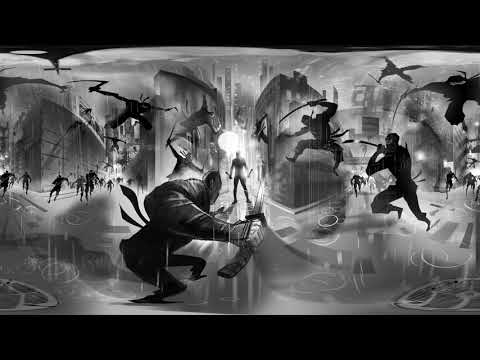The artwork is a vertically oriented, rectangular digital painting reminiscent of a comic strip, with prominent thick black horizontal stripes across the top and bottom. The scene is rendered in various shades of gray with touches of black and white, evoking a somber, rainy atmosphere, highlighted by swirling lines indicating rain and what appear to be puddles on the ground.

Set against a backdrop of towering, monochromatic skyscrapers in a cityscape, the artwork features multiple instances of the same ninja-like figure dressed entirely in black, wielding a long sword. This central character is depicted dynamically—leaping, crouching, and running across different parts of the scene, conveying intense action. In the middle background stands a formidable, larger antagonist—suggestive of a boss fight in a video game—also armed with a sword and rendered in light gray, commanding attention as the primary focus.

Additionally, the image includes various other figures—likely fellow combatants or additional ninjas—engaged in battle, some flying through the air with their swords, others positioned on the ground or making their way into the fray from the left side. One particularly noticeable figure, positioned in the lower left quadrant, is shown gripping a knife, his elbow prominently depicted close-up. The dynamic composition and atmospheric elements together create a vivid and dramatic scene, drawing strong visual parallels to the stylized aesthetics seen in the Sin City films.